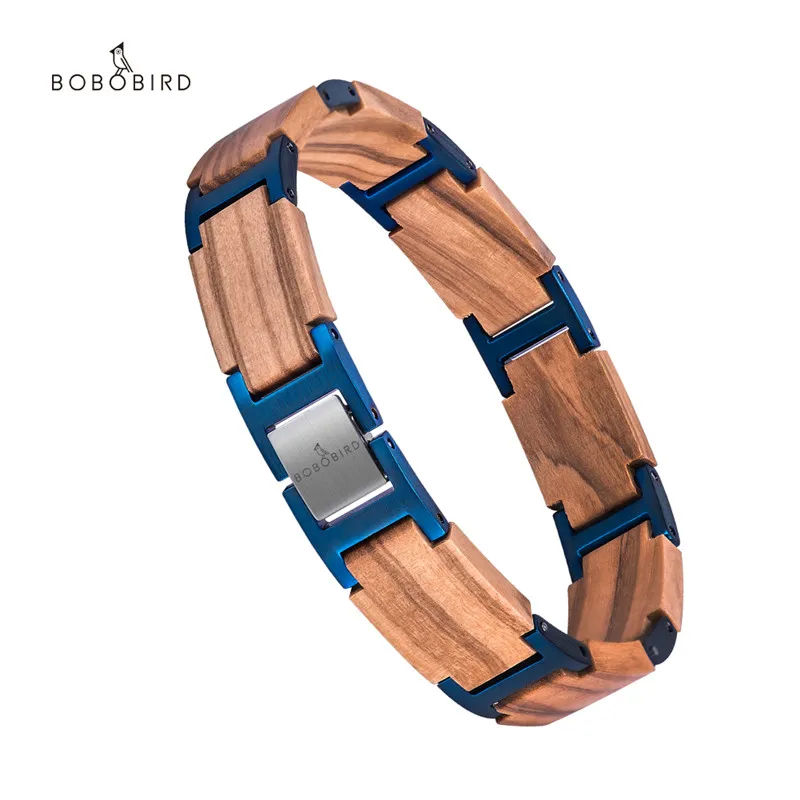The image features a product against a white background, prominently displaying the brand "BOBO BIRD" in black, all-capital letters at the top left corner. Above the text, there is a small bird icon perched on the second 'O' of "BOBO." The main focus of the image is a bracelet positioned diagonally. This bracelet is primarily composed of seven tannish medium-colored wooden links, showcasing visible wood grain with darker brown lines. These wooden pieces are interconnected by metallic blue aquamarine links resembling an I-beam structure. The bracelet is secured by a stainless steel clasp, which is silver and engraved with the "BOBO BIRD" name and the bird icon.